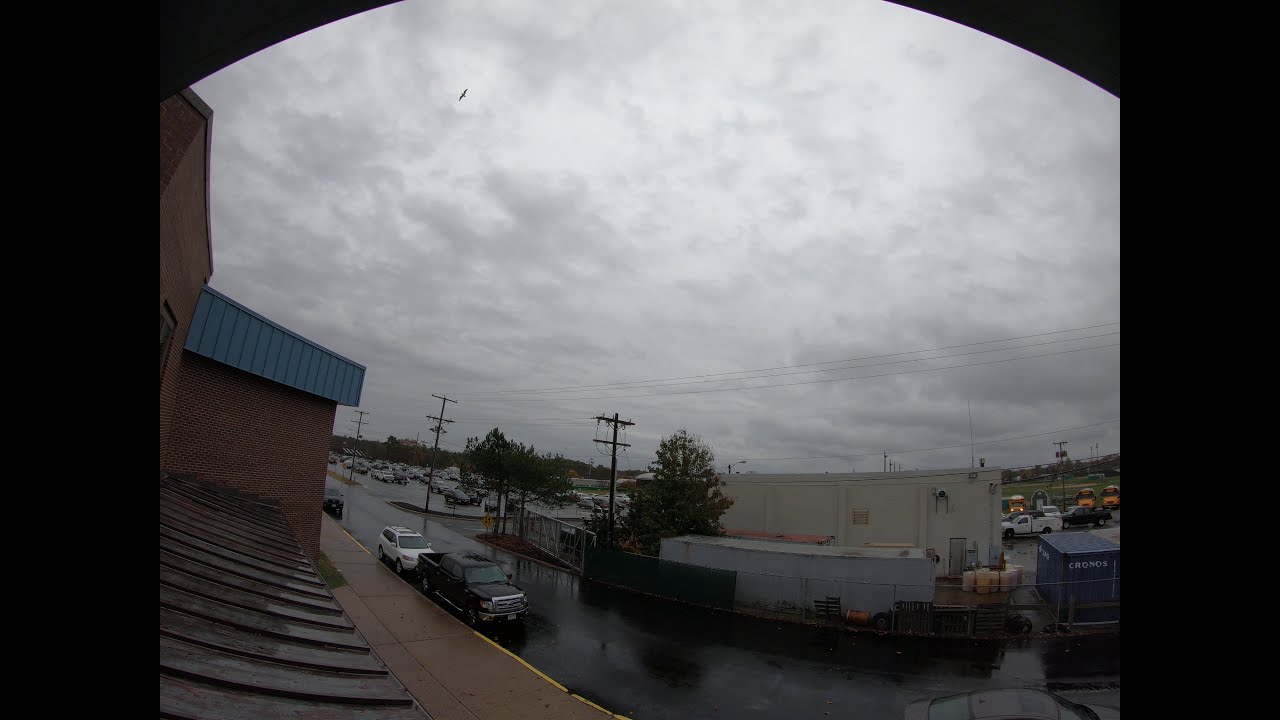The security camera image captures a large parking lot and the front road of what appears to be an industrial-like building. The overcast sky is dominated by dark and light gray clouds, suggesting an imminent rainstorm, with a solitary bird centered in the sky. On the left side of the image, there is a tan brick building with a light blue roof. The sidewalk in front of this building features a curved yellow marking, with a black pickup truck parked at the curb, followed by a white van. Towards the center, there is a white rectangular building adjacent to a blue shipping container. In the parking lot, various vehicles are visible, including school buses. The scene is further detailed by the presence of fencing and telephone wires crossing through the image, indicating an outdoor, industrial setting on a cloudy day.